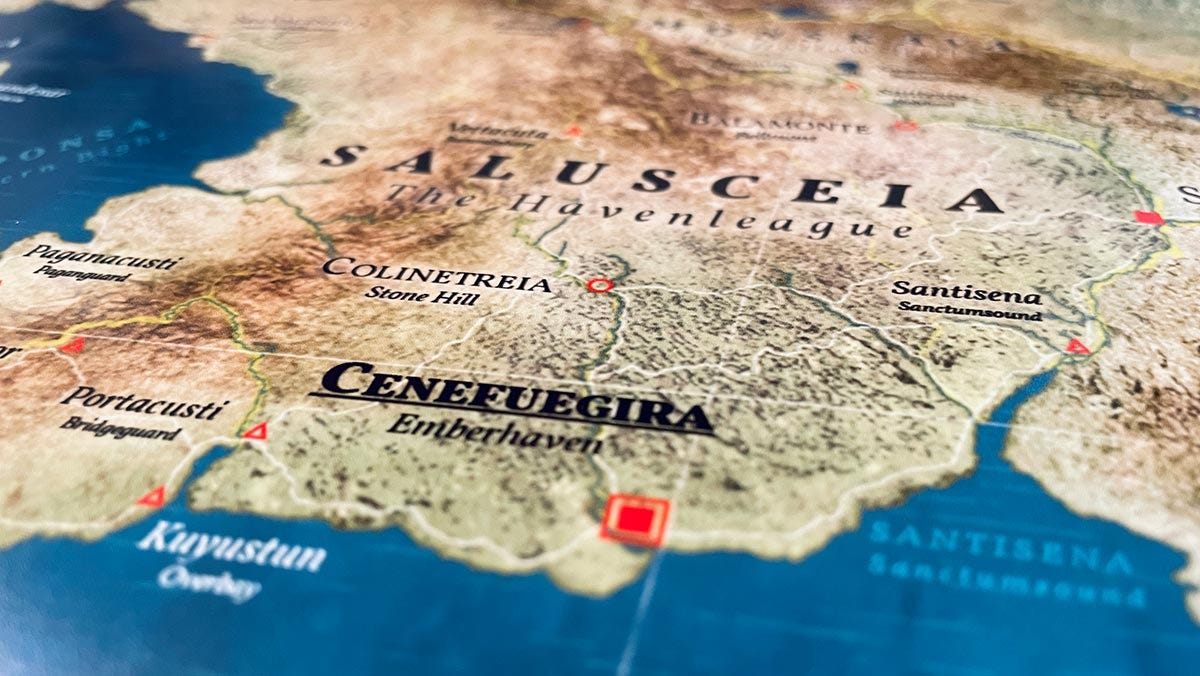The image is a color photograph of a detailed map taken at an angle, showing a flat, richly illustrated depiction of a land body surrounded by an ocean. The center of the map prominently features brown and green terrain, bisected by rivers denoted with blue squiggly lines. The largest black text in the middle of the land mass reads "Saluxeia, the Haven Lake," while below it, other areas such as Atreia and Forguera are marked. Surrounding this central land mass is a blue ocean, primarily occupying the bottom and partially extending to the upper left. In the ocean, names and details are printed in white and light blue text, identifying areas like Cayustan and Overbay.

Additional topographical features include a mountain range on the left side of the map. Various other locations are marked with red triangles, circles, and squares—details that add to the rich, descriptive nature of the map. Notably, a place marked with a square is named Senefuedjira, while another, marked with a triangle, is called Sentesena. The map also bears some semblance to the layout of Europe in its design, adding a layer of familiarity to its fantasy geography.